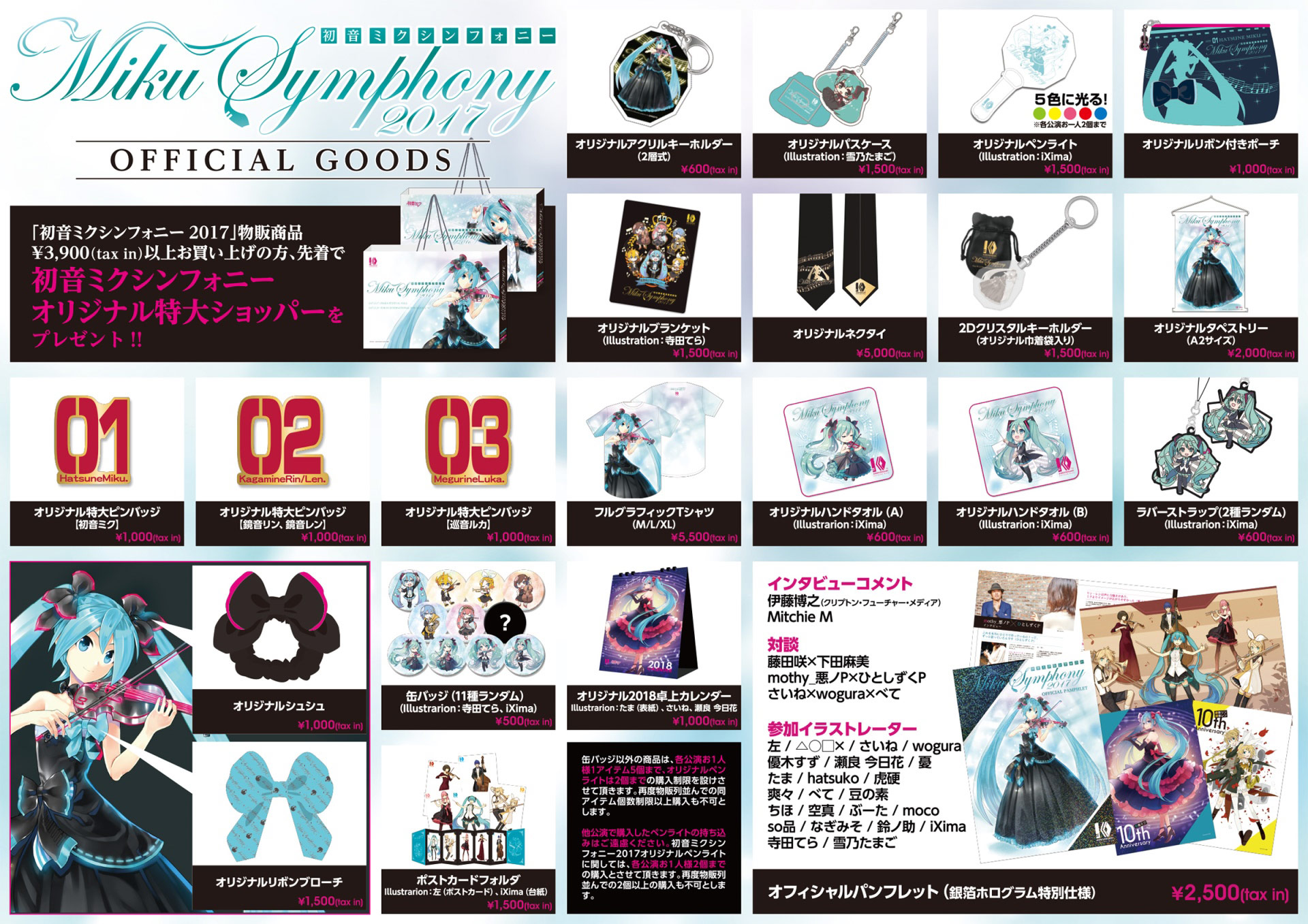The image showcases a vibrant assortment of official goods from the Miku Symphony 2017, featuring both English and Asian text. Prominently displayed at the top, the banner announces "Miku Symphony 2017 Official Goods." Among the diverse items, there are several anime-themed collectibles, including charms, keychains, earrings, and illustrations. Key products spotlighted include a tie with a rabbit or anime character, pins or badges with various anime designs, and two decorative bows—one black and pink, the other teal with black polka dots. The items are scattered throughout the image, simulating a catalog layout. Noteworthy items include a Miku Symphony 2017 Official Goods Calendar priced at ¥3,900, character images of Atsunamiku and Kagamine Len each for ¥1,000 plus tax, and a violin-playing anime character in a black and teal dress. The background colors are primarily white, light blue, black, hot pink, and peach, with occasional red and orange accents. This visually rich display, complete with intricate anime illustrations and memorabilia, encapsulates the essence of a shopping catalog or magazine dedicated to Miku Symphony merchandise.